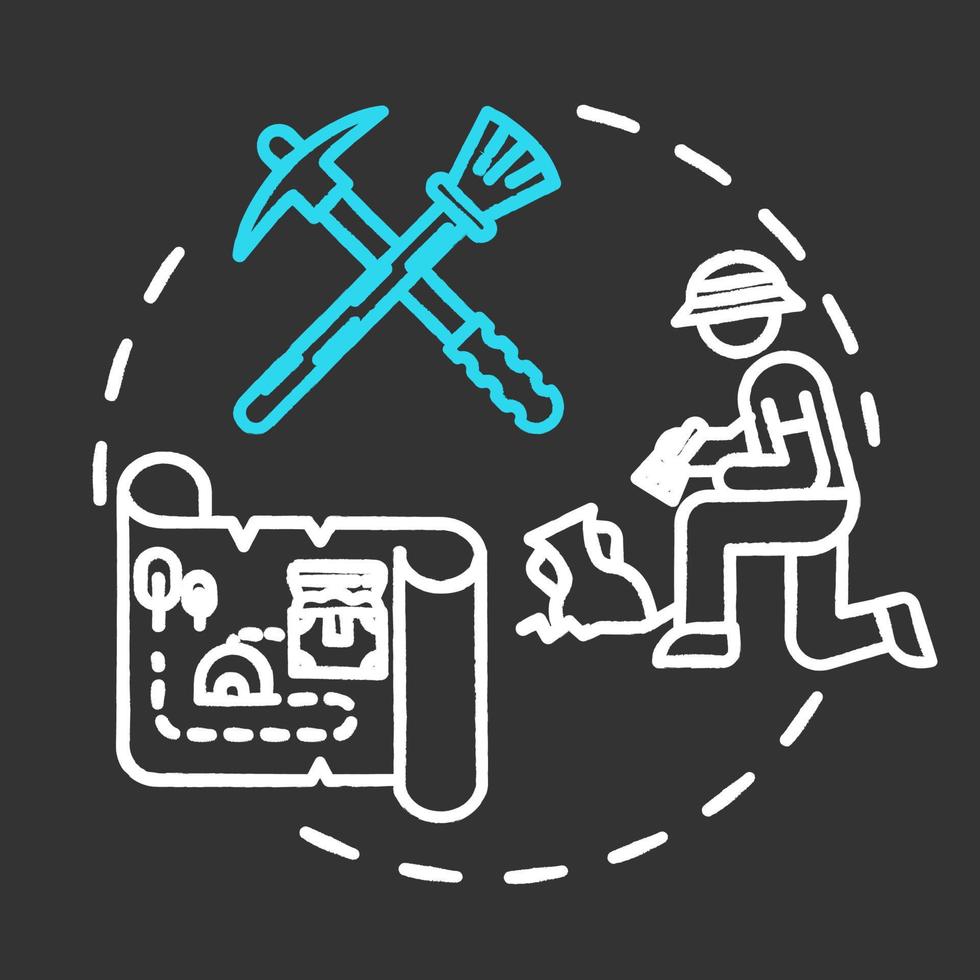This is a detailed illustration depicting what appears to be the entrance marker to an archaeological dig site. The image features a simply drawn, semi-stick figure person who has some body to it, bending on one knee with tools in hand, likely a pickaxe and a brush. The individual is digging up a vase that is partially buried in the ground. Surrounding the figure is a larger circle with small spaces in between, adding to the sign's structured yet straightforward design. Additionally, an illustrated map is visible, emphasizing the site's geographical and historical significance. The drawing serves as a visual indicator, warning passersby that excavation work is in progress and to be cautious of the area and the artifacts being uncovered.